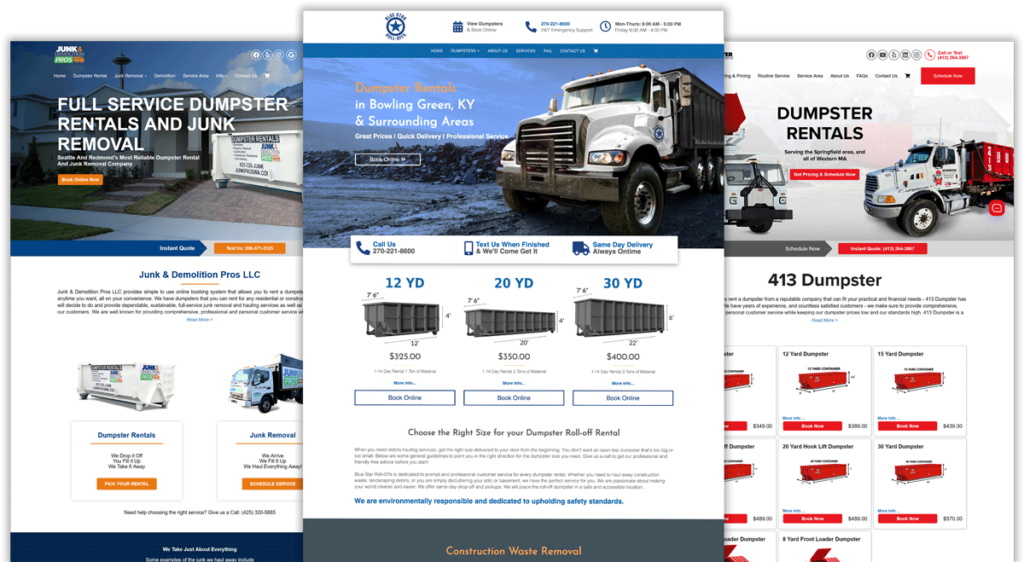The image showcases three different webpage examples, each dedicated to dumpster rentals and junk removal services.

**Left Webpage:**
- **Top Section:** Features a picture of a white house with a manicured green lawn, a white sidewalk in the foreground, and a light blue sky in the background. Overlaid in white text, it reads: "Full Service Dumpster Rentals and Junk Removal."
- **Middle Section:** Displays the company name, "Junk and Demolition Pros LLC," in green text against a white background.
- **Bottom Section:** Shows two columns with headers. The left column reads "Dumpster Rentals" and the right column reads "Junk Removal." Below these headings, there is an image of a large dumpster and a trash truck.

**Right Webpage:**
- **Top Section:** Contains two images of trucks on a white background. The left image features a large truck with a dump bed, while the right image shows a white truck with a red cart in the back. The title "Dumpster Rentals" is displayed in black text at the top.
- **Middle Section:** Labeled "413 Dumpsters" in black text, featuring a grid of nine squares each displaying red containers with dimensions and price tags underneath.

**Middle Webpage:**
- **Top Section:** Highlights a white truck with a large black container in the back. In the center top, it reads: "Dumpster Rentals in Bowling Green, Kentucky, and Surrounding Areas."
- **Bottom Section:** Includes three images of gray containers of varying sizes, labeled 12 yards, 20 yards, and 30 yards from left to right. Below each container, the respective prices are listed as $325, $350, and $400. Additional text appears below the images, providing more details. 

These detailed web pages offer a comprehensive look at dumpster rental and junk removal services with clear imagery and informative layouts.